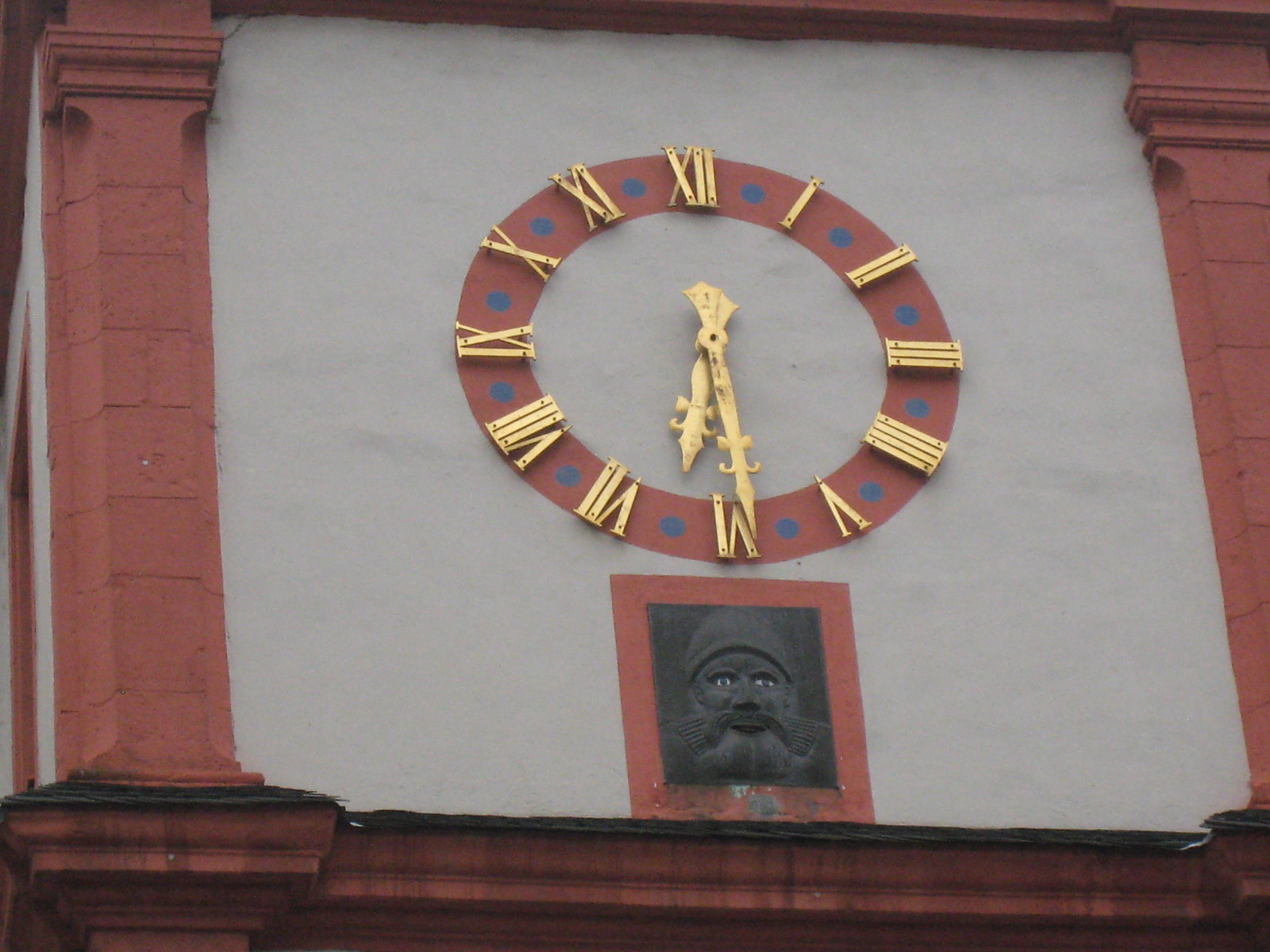The image is a slightly rectangular, horizontally-aligned frame capturing an upward view of a portion of a building. Dominating the composition are two prominent, rusty red columns positioned symmetrically on the right and left sides. Between these columns, the background is a pristine white, drawing attention to the central elements. In the middle of the image, there is a striking red circle with an open center, allowing the white background to remain visible through it. This red circle is adorned with gold Roman numerals and gold clock hands, clearly indicating it is a clock. Beneath the clock, within a red square border, is a detailed black sculpture of a face, adding an artistic touch to the architectural scene.